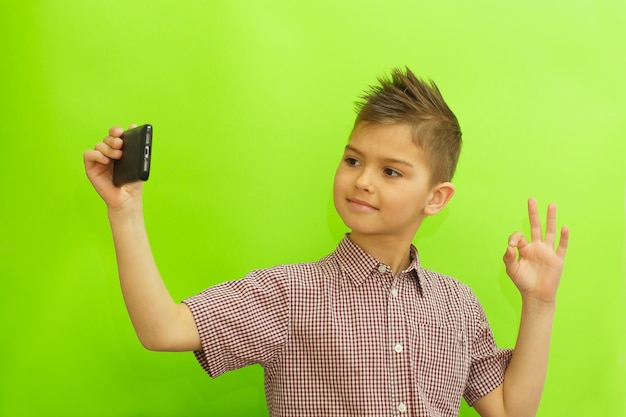The image is a horizontal rectangular photograph of a young boy, primarily visible from his lower chest up to his head, set against a solid bright lime green background. The boy, standing slightly off-center towards the right, wears a short-sleeved plaid collared button-up shirt with white plastic buttons, the top button undone, and a chest pocket on his left side. His hair is styled in a gelled-up manner reminiscent of a mohawk, with shorter sides. He appears to be smiling as he holds a black cell phone in his right hand, tilted sideways towards the upper left, possibly taking a selfie. His left arm is bent at the elbow, raised up to display an OK sign with his thumb and index finger forming a circle and the other three fingers extended. The vivid and varied colors in the image include green, black, silver, gray, peach, tan, and red.